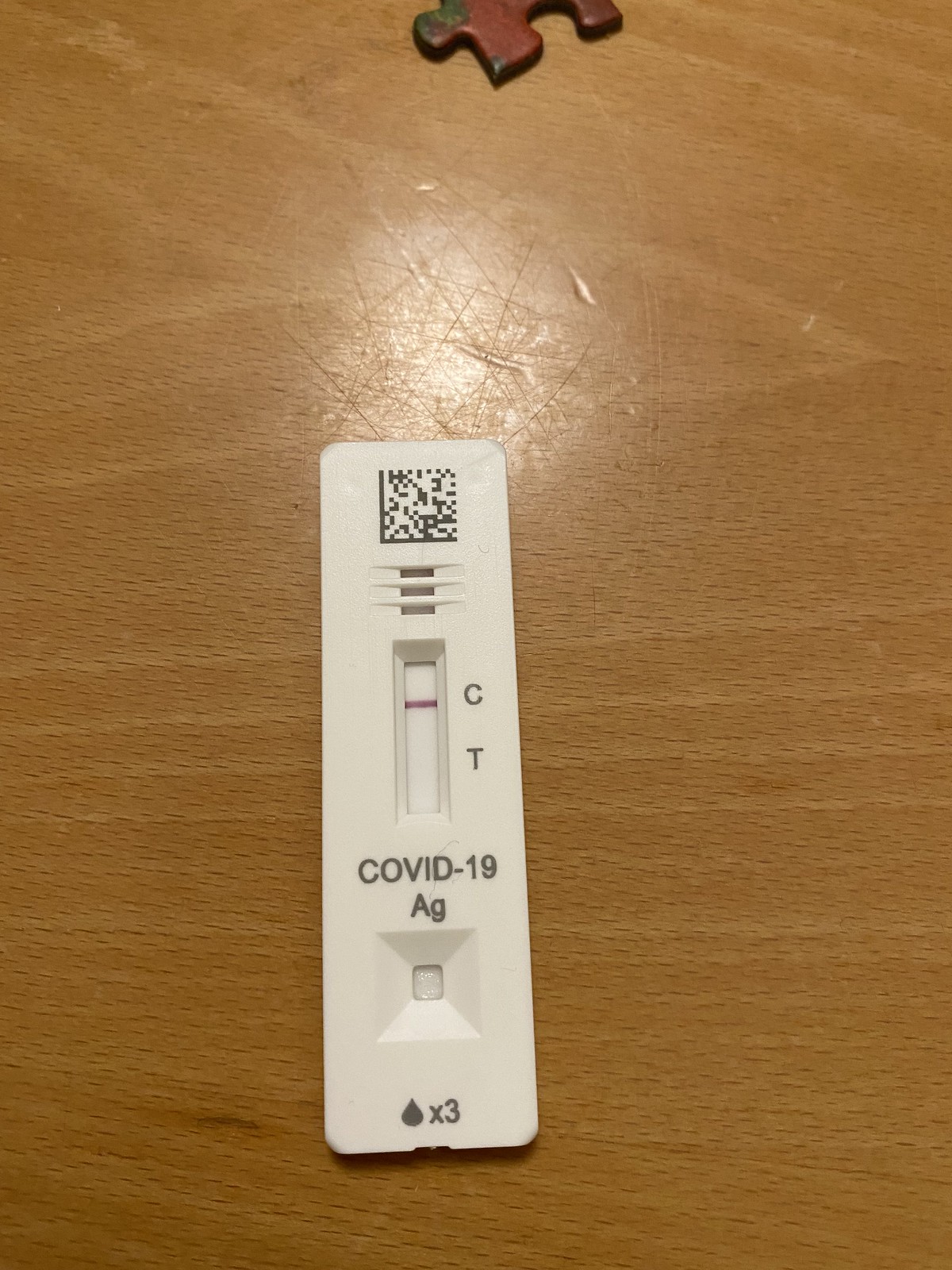This portrait-format photograph captures a COVID-19 test resting on a golden brown table or countertop. At the top of the image, a single puzzle piece is discernible. This piece, showing a circular head and a part with one hole for connection, features a maroon color on the legs and a hint of dark green towards the round head. The scene is illuminated by an overhead light, casting a gentle glow on the table's surface.

Prominently positioned in the lower middle section of the picture is a white plastic COVID-19 test resembling a pregnancy test kit. At the top of the test, a scannable barcode is visible, likely for identification or result retrieval purposes. Below the barcode are three small holes, followed by a long rectangular window. Within this window, a thick red horizontal stripe next to the letter "C" indicates a control line. Lower in the window, the letter "T" is noted, which would show if the test is positive when a second stripe appears. 

Beneath the window, the inscription "COVID-19 AG" is printed, indicating the test type. Further down, a small square likely serves as the area where a sample, such as blood, would be applied. At the test's base, a small droplet icon is present next to the instruction "x3," indicating the necessary amount of liquid needed for the test. The overall composition gives a detailed view of the testing device in a calm, neutral setting.